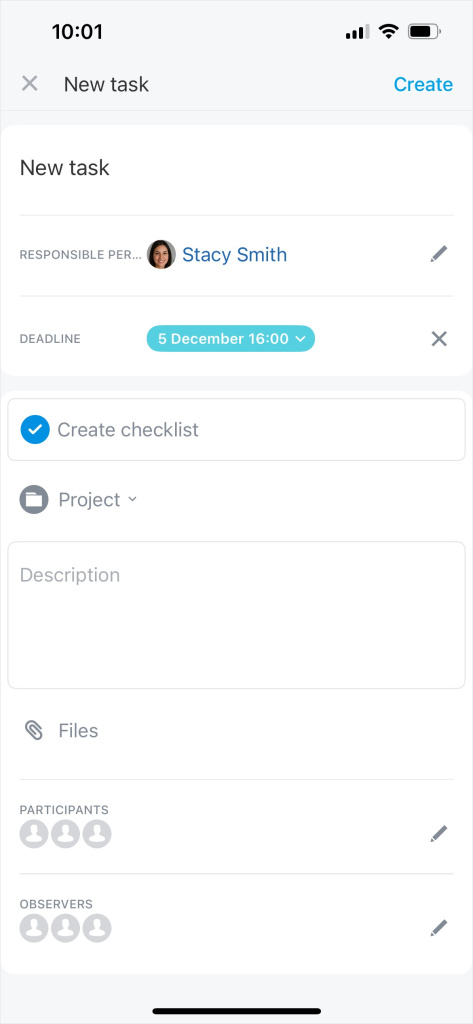The image is a vertically oriented screenshot of a mobile phone interface with a white background. A wide, light gray banner at the top displays the time, "10:01," in the left-hand corner and various icons in the right-hand corner. Below this banner, the header reads "New Task" with an "X" to its left and "Create" in blue font to its right.

Further down, the text "New Task, Responsible Person" is displayed alongside a circular portrait icon with "Stacy Smith" highlighted in blue. A pen icon is located on the right side, indicating an option to edit. Below this section, a blue bar marked with "5 December 16:00" features a drop-down menu and an "X" to the right.

Following this, a section labeled "Create Checklist" appears, featuring a white check mark within a blue circle. Adjacent to this is a file icon labeled "Project." An empty description box sits underneath. The "Files" section, marked by a paper clip icon, is found below the description box. Two subsequent sections labeled "Participants" and "Observers" include pencil icons on the right, also implying edit options.

A thin black horizontal line marks the bottom of the image, completing the layout.